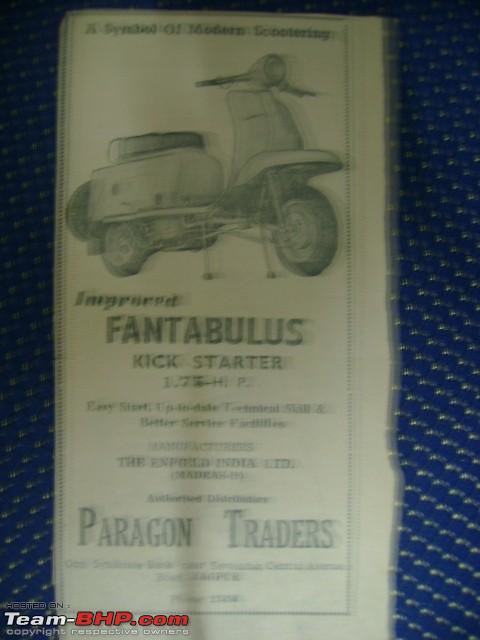A color photograph features an old black-and-white newspaper clipping of a scooter advertisement, with a blue fabric background adorned with white polka dots, possibly from a couch cushion. The ad, titled "Improved Fantabulous Kickstarter 1.75 HP," is slightly out-of-focus, making some of the text underneath hard to read. It clearly mentions "The Enfield Indian" and "Paragon Traders." The scooter, which appears to have three wheels (two at the back and one at the front), stands on a kickstand, with a large headlight attached to the handlebars and a cushioned seat offering storage underneath. At the bottom right corner, there is a watermark that reads "TEAM-BHP.com copyright respective owner."